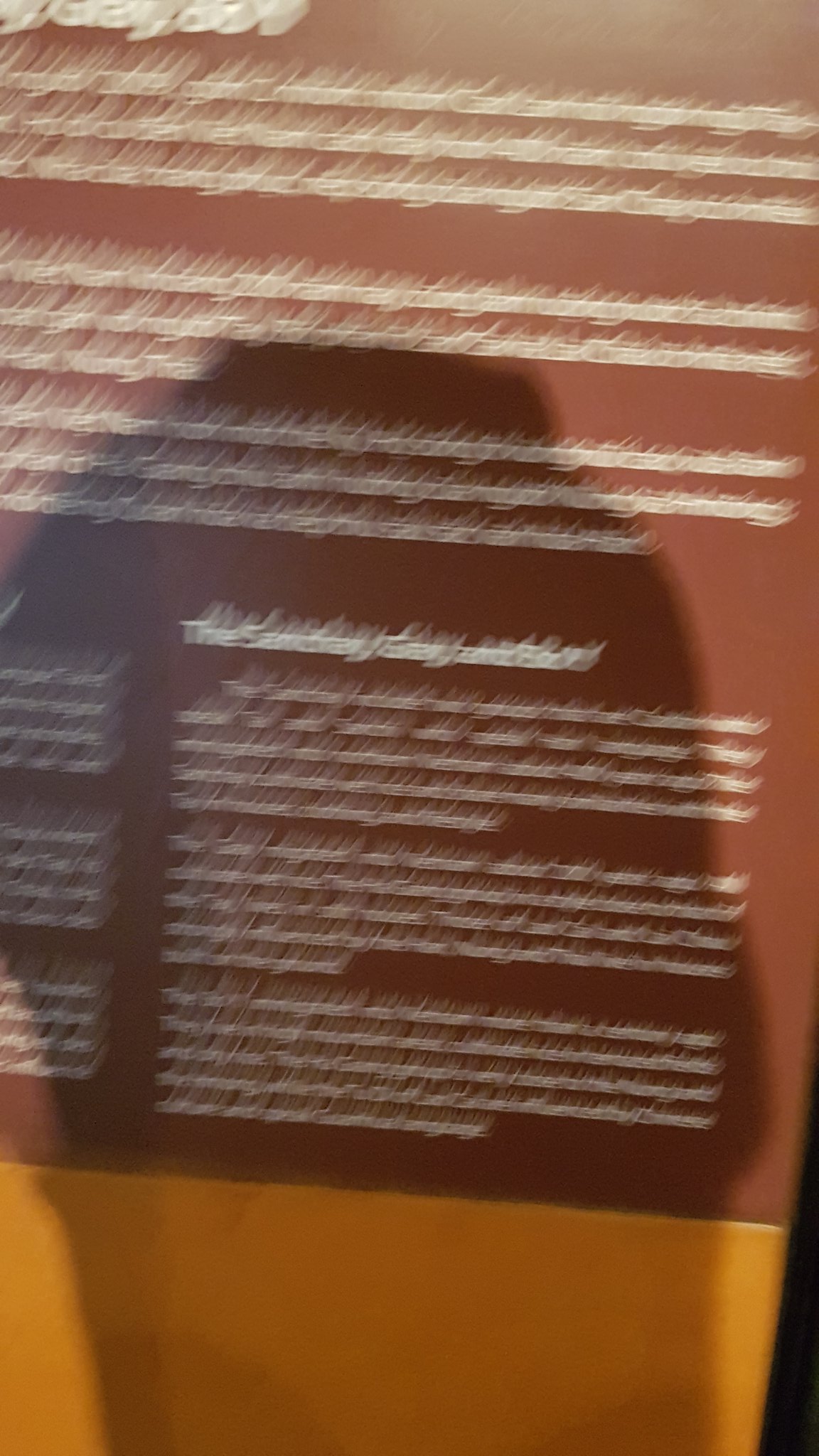This low-resolution, blurry image features a board with text that is difficult to discern due to the poor image quality. The board is divided into two sections: the top part is dark brown while the bottom part is orange. The text on the board is white, but it remains illegible due to the fuzziness of the image. A small black patch is visible in the bottom right corner of the board. Additionally, a shadow appears across the middle of the board, further obscuring the details.